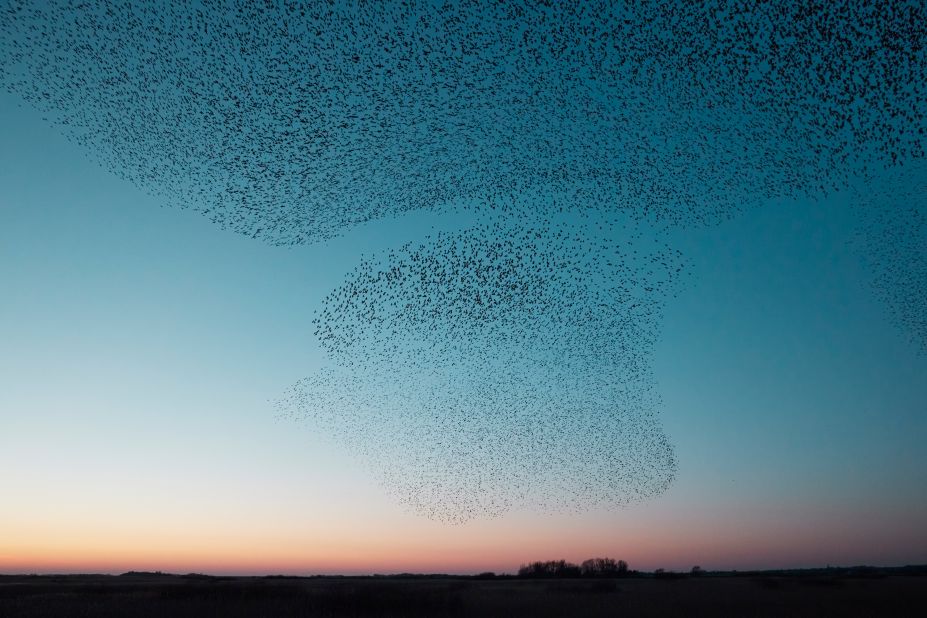In this photograph taken in an outdoor natural setting during the evening, the bottom displays a dark, somewhat obscure ground, hinting at the advancing dusk. Above, an expansive sky transitions dramatically in color, from a deep blue at the top to a gradient of yellow and pink mid-sky, culminating in a reddish hue near the horizon. Dominating the sky is a striking formation of birds, their dense, black silhouettes creating a mesmerizing, tornado-like pattern. The birds are primarily concentrated toward the top right, where they form a wide array, slightly dispersed but still maintaining a circular, cyclonic appearance as they seem to swirl and approach the viewer. The clear, vivid skyline juxtaposed with the dark, dynamic shapes of the birds adds to the dramatic and almost surreal quality of the scene.